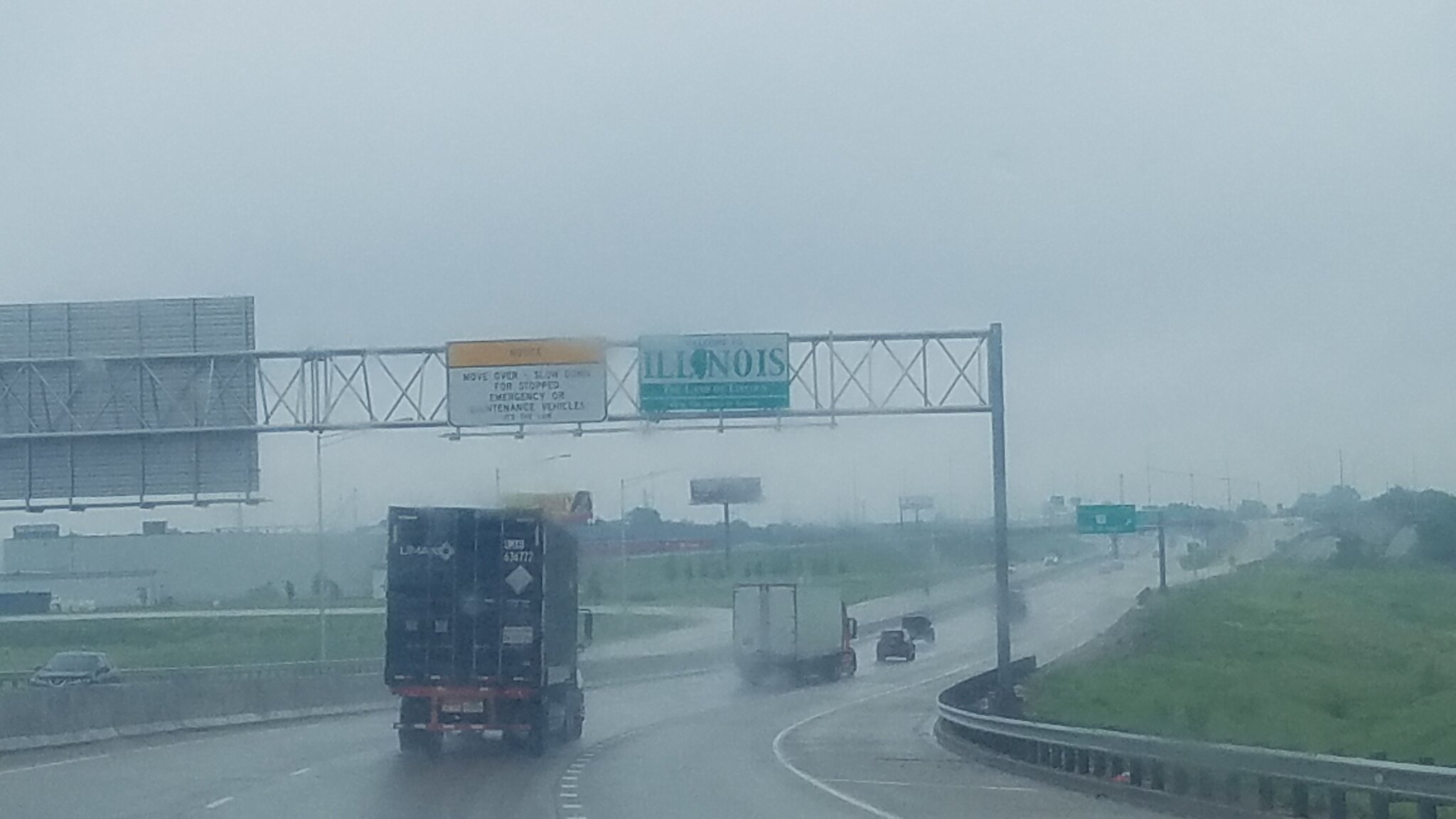The image is a detailed, hazy photograph of a highway on a rainy and foggy day, appearing to be taken from the right-hand lane. The highway stretches through green, mowed plains of grass on either side with patches of green and gray spots scattered across the scene. Dominating the foreground are two semi-trucks, a black one closer to the camera and a white one further away, along with a few regular vehicles including two black cars. Above the road, a metal structure supports several signs: a prominent green one reading "Welcome to Illinois," signifying the crossing into Illinois, and another white and yellow notice advising drivers to "Move Over, Slow Down for Stopped Emergency or Maintenance Vehicles." The sky is a hazy, bluish-gray, blending with the fog that obscures the distant power lines, billboards, and additional highway signs further down the road.